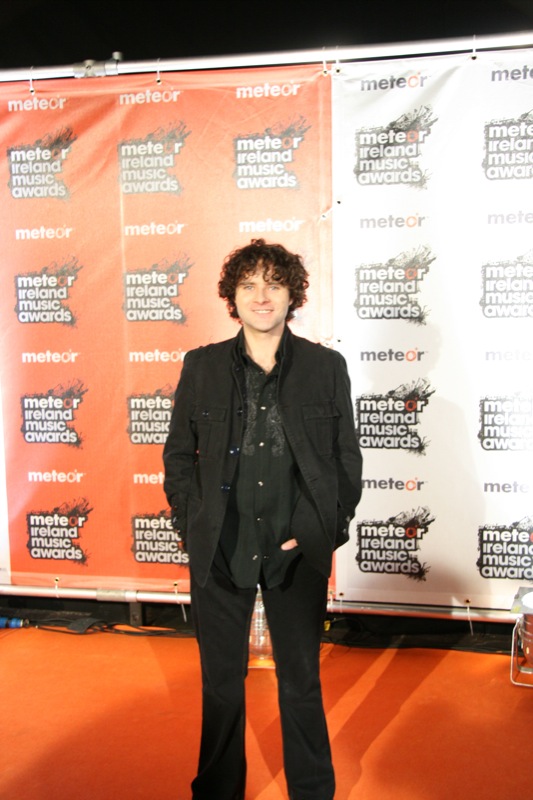A man, dressed in an all-black ensemble featuring black pants, a black button-down shirt, and a black jacket, is standing on an orange carpet at the Meteor Ireland Music Awards. He has curly brown hair and is smiling, with his hands casually placed in his pockets, one finger notably sticking out. Behind him is a promotional backdrop for the event, symmetrically divided into an orange section on the left and a white section on the right, both displaying the text "Meteor Ireland Music Awards" in white letters outlined in black. The man faces the camera with a slightly awkward stance, giving off the appearance of a typical red-carpet photo.